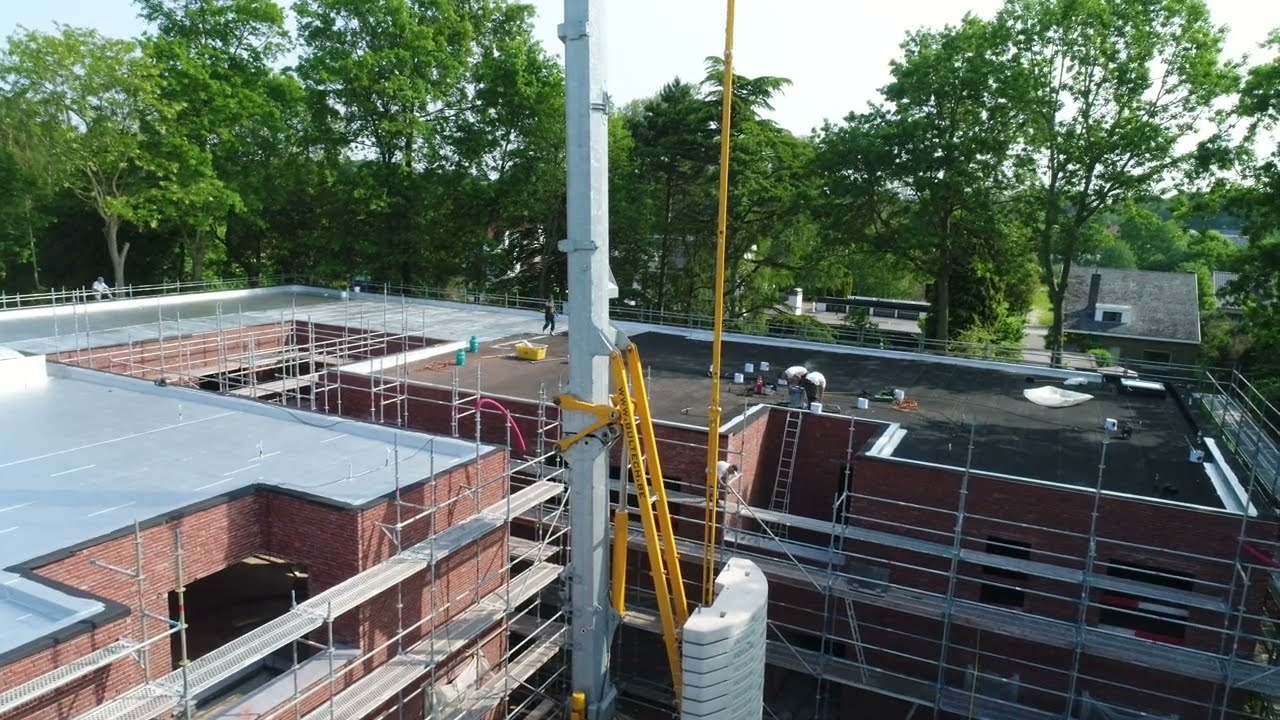The image depicts the overhead view of a construction site focused on an incomplete flat roof of a red brick building, flanked by extensive scaffolding. Workers in dark clothing and white shirts are concentrated on the black-colored section of the roof, bent over and engrossed in their tasks. The rest of the roof sports a silver hue. Prominently featured in front of the building is a complex structure that includes a large silver pole connected to a yellow ladder, with a white weight barrier at its base and a long yellow pole extending from its top, bearing the text "www.boldtech.be." The background showcases green leafy trees and distant buildings with gray roofs, one of which includes a large chimney and a white attic outlet. The skyline above the trees is primarily white and hazy, enhancing the industrial atmosphere of the scene.